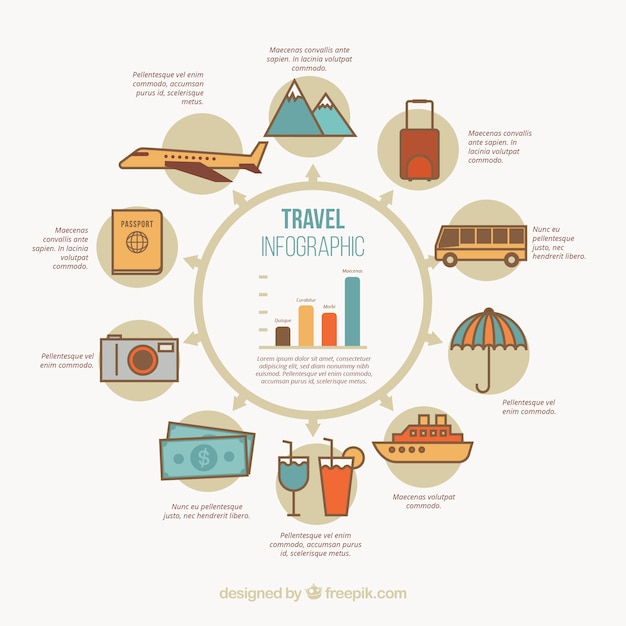The image is a travel-themed infographic with a central brown circle outline that contains the text "travel infographic" in blue. Below this title is a bar graph, but the text under the bars is not clearly legible and appears to be in a non-English language, possibly Latin. The bar graph consists of four vertical bars of different colors and heights: the tallest bar is blue, followed by a tan bar, an orange bar, and finally a shorter brown bar.

Surrounding the central circle are small, colored circles each containing different travel-related icons. At the top is an image of mountains colored blue, symbolizing outdoor adventures or destinations. Clockwise from the top, the next icon is a brown suitcase, indicating travel luggage. Following that, a red bus represents transportation, a purple umbrella signifies beach destinations, and a green cruise ship is for sea travel or cruises. There are also two blue drinks suggesting leisure or nightlife, green money implying expenses or budget, a yellow camera for photography, a red passport representing travel documentation, and a large blue plane indicative of air travel. Each icon is paired with text that is not in English and is difficult to decipher. At the bottom of the graphic, the credit reads "designed by freepipe.com."